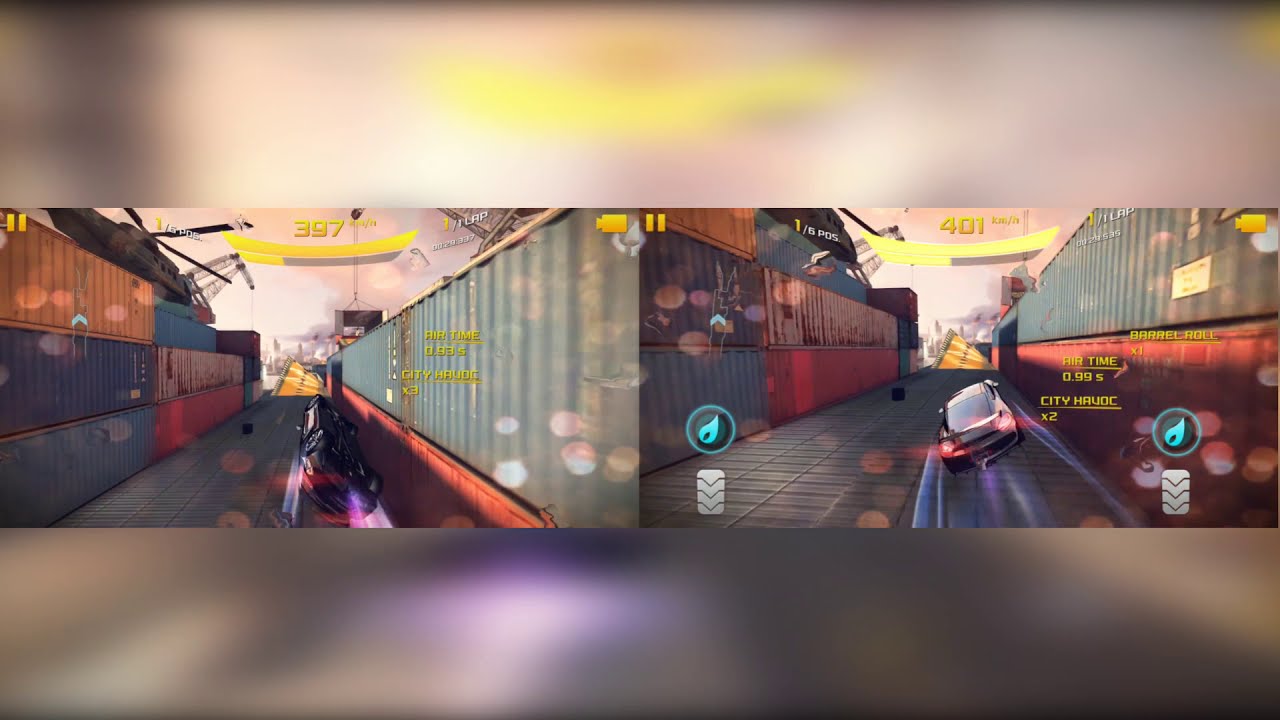The image captures two distinct yet nearly identical screenshots from a third-person racing video game, arranged side-by-side. Both screenshots showcase a car racing through a shipping container field configured like a hallway, leading up to a yellow ramp that seems poised for a jump. The first panel on the left shows a car in mid-air, performing a spiral trick against the backdrop of container walls and a visible speedometer at the top. The second panel on the right depicts a different car, no longer in mid-air but navigating the same corridor with its brake lights illuminated. The background includes additional elements like a helicopter and crane on top of the shipping containers and a hazy sky. The entire composition is bordered by blurry, colorful rectangles above and below, dominated by hues of yellow, black, purple, white, and gray.